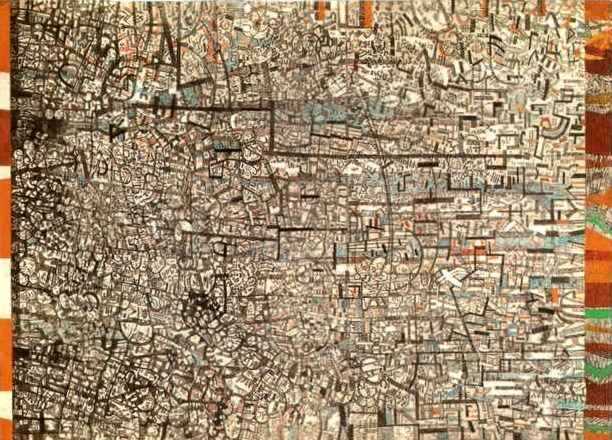The image depicts a highly intricate and busy artwork that resembles an aerial view of a sprawling city filled with buildings and an extensive network of roads. The main design, primarily in shades of black, white, and gray, mimics the intricate layout one might observe from high above. Small specks of orange, dark reddish-brown, and pastel blue add subtle color variations throughout the central area. On the left and right edges, the artwork features distinct pattern strips with vibrant hues of orange, red, yellow, and cream, which may suggest borders or a framing element. The entire composition evokes the complexity of a cityscape, likened to a mosaic map without text, where one could imagine streets and homes embedded within the chaotic but beautiful design. This piece, combining the aesthetic of aerial imagery with the texture of fabric or table setting, would make a striking addition to a minimalistic decor, such as a bedroom or foyer wall.